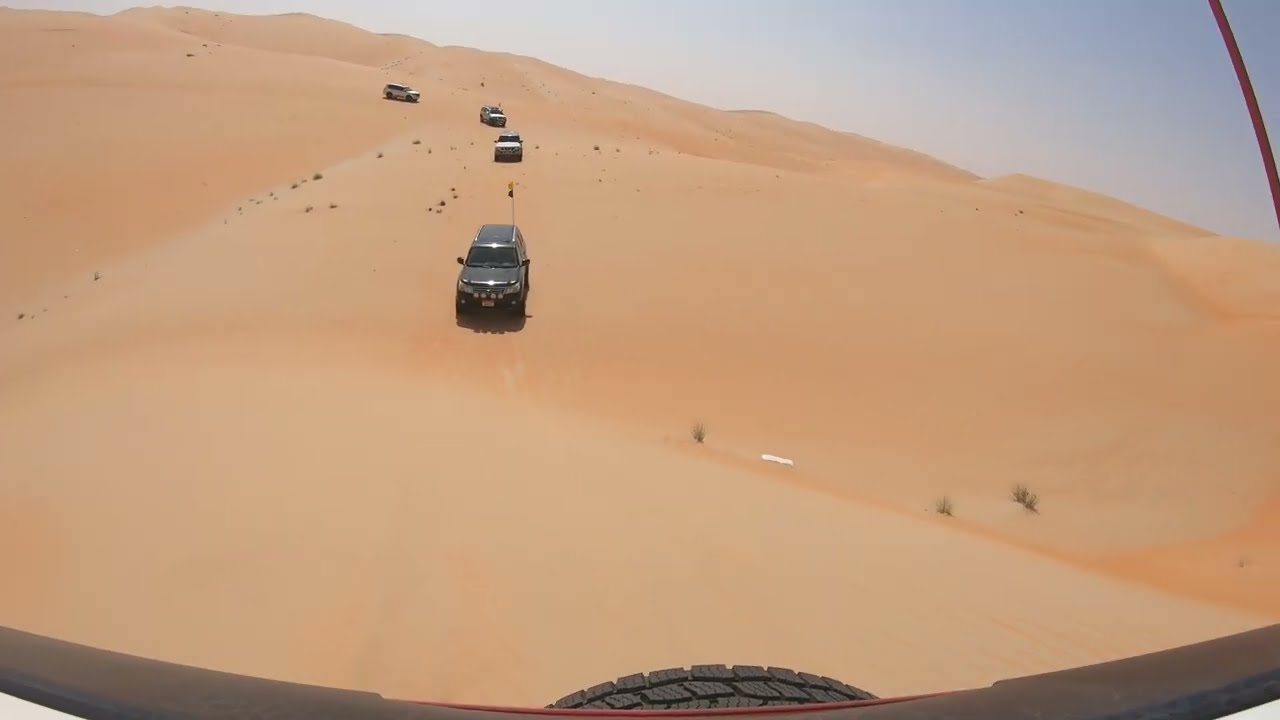In the midst of a vast, sandy desert, a procession of five SUVs traverses the rugged terrain. The lead vehicle, a gray van adorned with a small flag on its front pole, commands the convoy, with four other vehicles trailing behind in a straight line. Among the followers, a white SUV brings up the front, followed by another gray car, and two more white cars completing the formation. The desert landscape is punctuated by small greenish-brown plants, possibly cacti, scattered across the expansive sandy dunes. The image seems to be captured from the perspective of the rear of the leading vehicle, as indicated by a spare tire visible at the bottom of the frame. The sky occupies the upper portion of the image, adding a vast, open feel to the scene in the middle of the day. The vehicles tread a largely pathless expanse, highlighting the raw, natural beauty of the desert setting. The predominant colors include sandy browns, greenish hues from the plants, grays, whites, and touches of black, reflecting an adventure in a minimalist yet striking landscape.